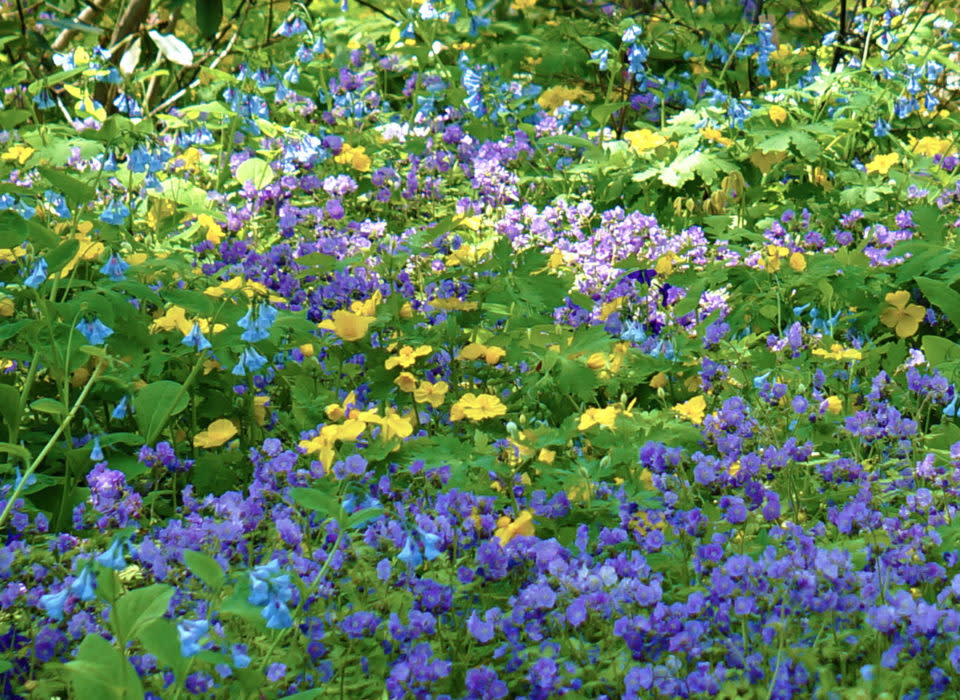This vibrant outdoor daylight photograph captures a riot of pastel-colored flowers in a lush, natural setting, likely a forest or wooded area. The scene is dominated by a thick scatter of small purple flowers, with additional clusters of light blue, yellow, and white blooms interspersed throughout. Green leaves and stems weave among the flowers, adding to the abundant foliage that occupies most of the image. In the far background, the photograph reveals tree trunks and more greenery, contributing to the sense of a dense, lively forest. The scene is brightly lit, suggesting a sunny, pleasant day, and the overall aesthetic is one of serene beauty and natural richness.